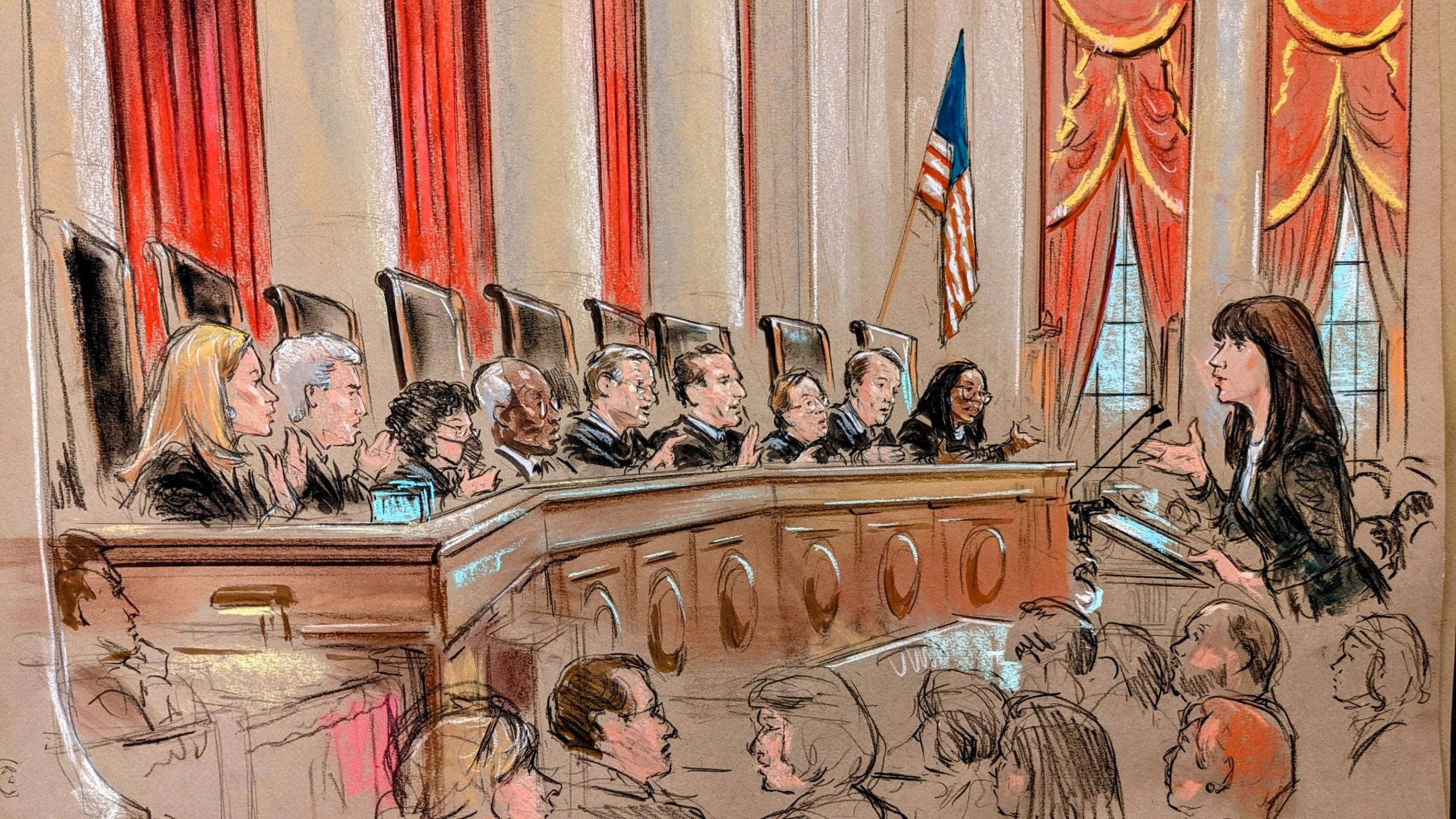The image depicts a detailed courtroom scene captured by a courtroom artist. On the left side of the artwork, a long, slightly curved bench features nine judges, all dressed in traditional black robes. Among them, the third judge is a woman wearing a black facial mask reminiscent of those used during COVID-19. Behind each judge are tall-backed black chairs, with an American flag prominently displayed on a flagpole centered behind them. The background showcases large windows adorned with red and brown drapery. 

In the foreground to the right, a woman in a black business suit, with long brown hair, stands at a podium equipped with microphones, likely addressing the court. Below her are several abstractly depicted faces suggesting audience members or jury participants. On the lower left, a person seated in what appears to be the testimony area contributes to the dynamic atmosphere of the scene. The overall color palette of the piece is dominated by muted browns and reds, lending a solemn, almost reverent tone to the depiction of this judicial setting.